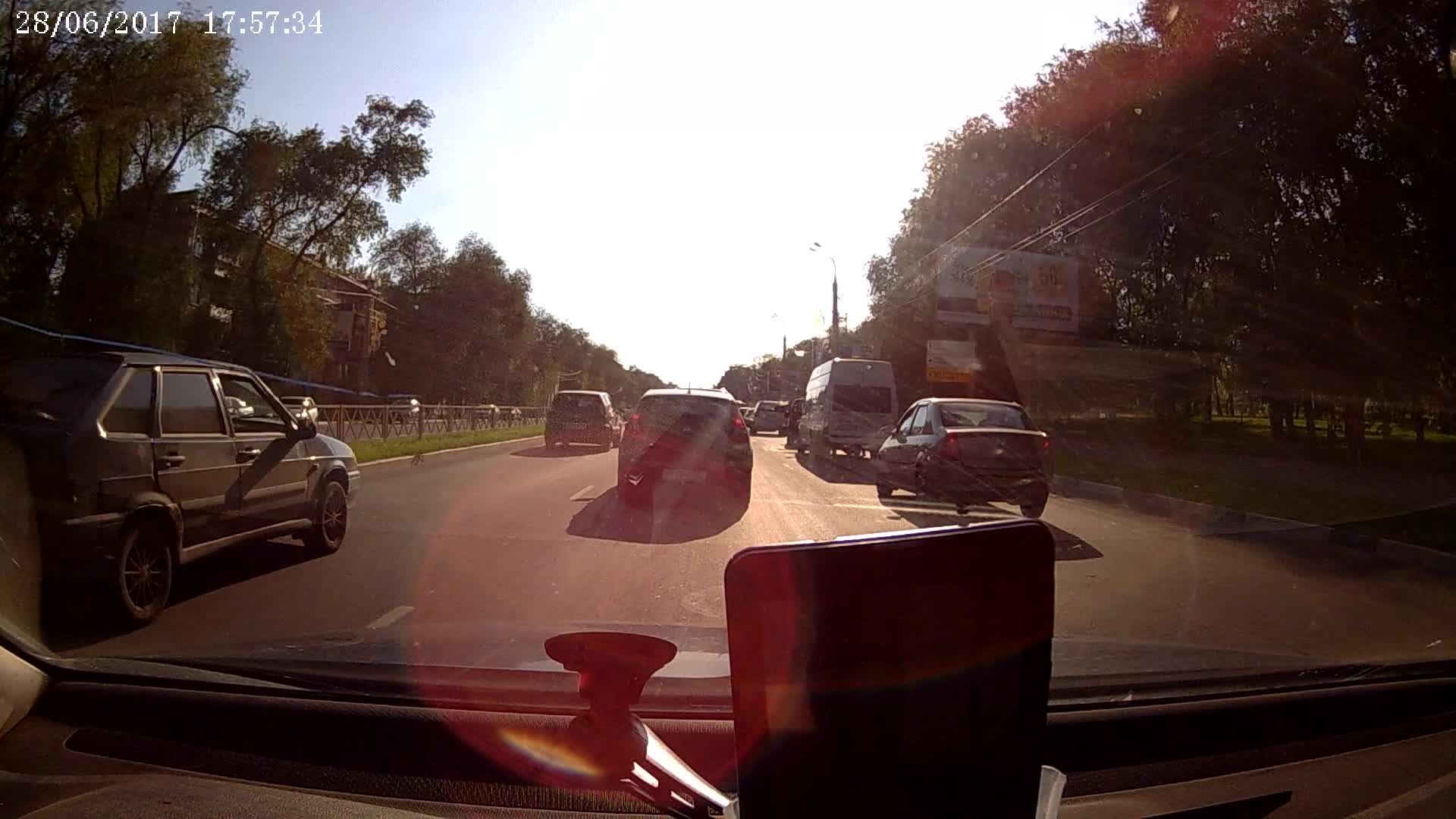The image captures a bright, sunny day from a first-person perspective, taken through the windshield of a car, suggesting it's from a dashcam. In the top left corner, the timestamp reads "2008, 06, 2017, 17:57:34". The road is a wide three-lane highway with a grassy median separating opposing traffic lanes. Trees with many green leaves line both sides of the road, with some wires visibly crossing overhead. On the left side of the image, there's a fence and possibly a building partially obscured by the trees. On the right, there is a strip of pavement alongside which a billboard stands. 

There are several vehicles ahead, including a blue or black front bumper of a car just in front, a black truck or SUV, and a white van. The sun, positioned directly ahead and slightly low in the sky, results in significant glare on the windshield and camera. The sky is clear and vividly blue. The image also shows some asphalt on the road and the top of a turned-off phone mounted on the dashboard, emphasizing the scene's POV nature.